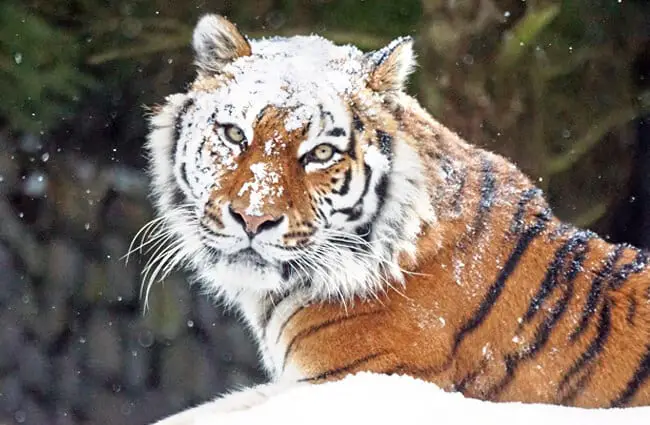The photograph captures a mesmerizing scene of a majestic tiger lying in the snow. The tiger, with its striking orange coat adorned with black stripes, has its head turned to the left, directly facing the camera. The image focuses on the tiger's face and the left side of its body, extending midway down its back, thus excluding the back legs and tail. The tiger's face, covered in a generous dusting of snow, gives the impression that it playfully buried its face in a snow pile. Snowflakes can be seen gently falling, enhancing the wintry atmosphere.

The close-up reveals the tiger's exquisite features: its piercing eyes exuding curiosity, long white whiskers, and a ruff around its neck and face. Black specks dot its cheeks, adding to its allure. Its ears, alert and cat-like, and the thin black stripes on its white face contribute to the tiger's magnificence. The background features a gentle snowfall, further blanketing the serene scene. Overall, the photograph beautifully encapsulates the tiger's regal presence in a snowy landscape.